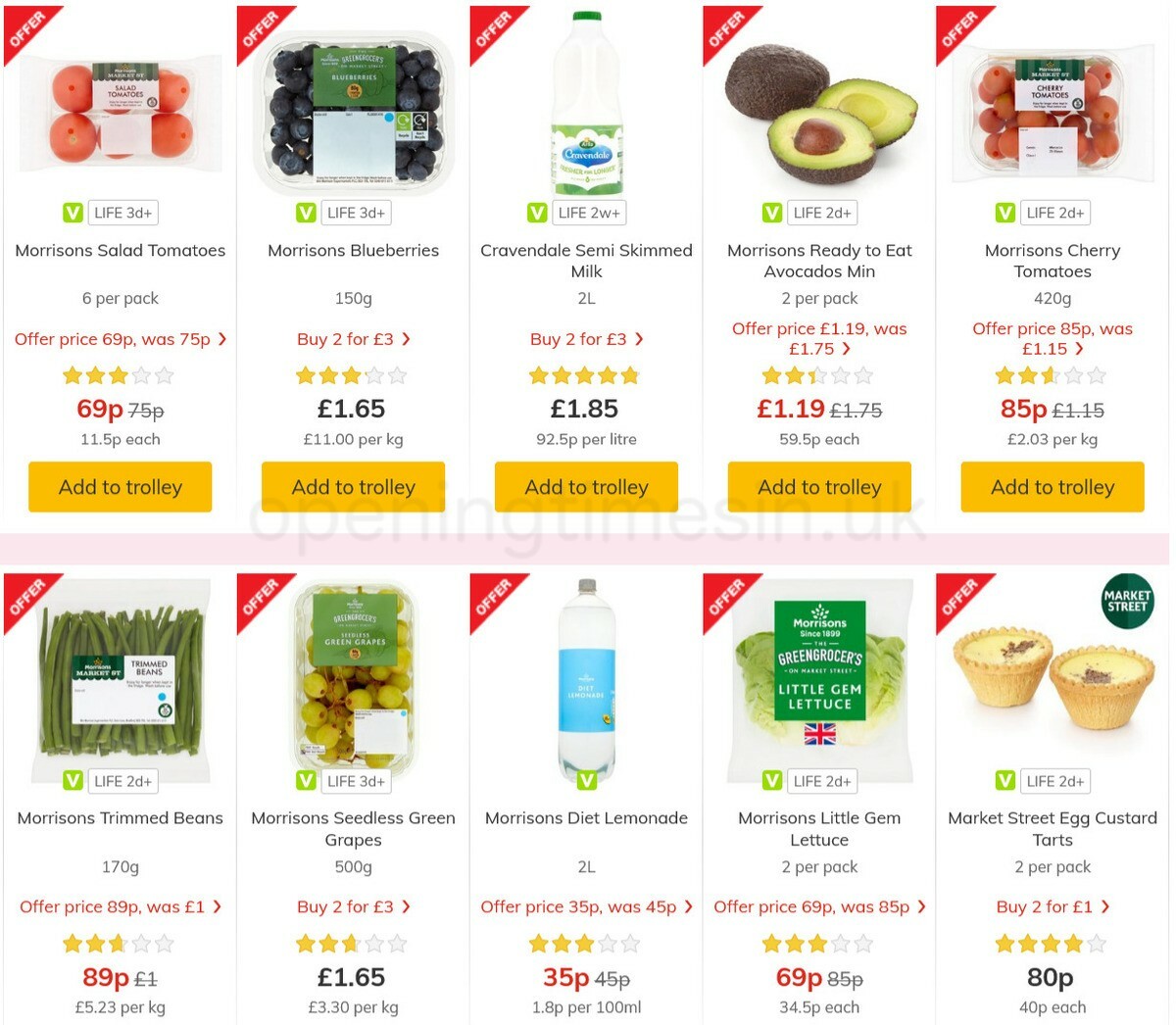**Detailed Description of Grocery Store Shopping Page Screenshot:**

The image is a screenshot of a grocery store's online shopping page, specifically Morrison's. The layout features two rows and five columns, showcasing a total of ten different food products. Each product is displayed within its own cell, which includes various details such as the product image, special offers, pricing, star ratings, and action buttons.

**First Row Products:**
1. Morrison's Salad Tomatoes
2. Morrison's Blueberries
3. Cravendale Semi-Skimmed Milk
4. Morrison's Ready-to-Eat Avocados (Minimum two per pack)
5. Morrison's Cherry Tomatoes (420 grams)

**First Row Offers & Ratings:**
- Morrison's Salad Tomatoes: Offer Price 69p (originally 25p), Rating: 3 out of 5 stars
- Morrison's Blueberries: Buy 2 for £3, Rating: 3 out of 5 stars
- Cravendale Semi-Skimmed Milk: Buy 2 for £3, Rating: 5 out of 5 stars
- Morrison's Ready-to-Eat Avocados: Offer Price £1.19 (originally £1.17.5), Rating: 2.5 out of 5 stars
- Morrison's Cherry Tomatoes: Offer Price 85p (originally £1.15), Rating: 2.5 out of 5 stars

**Second Row Products:**
1. Morrison's Trimmed Beans
2. Morrison's Seedless Green Grapes (500 grams)
3. Morrison's Diet Lemonade (2L)
4. Morrison's Little Gem Lettuce (two per pack)
5. Market Street Egg Custard Tarts (two per pack)

**Second Row Offers & Ratings:**
- Morrison's Trimmed Beans: Offer Price 89p (originally £1), Rating: 3 out of 5 stars
- Morrison's Seedless Green Grapes: Buy 2 for £3, Rating: 3 out of 5 stars
- Morrison's Diet Lemonade: Offer Price 35p (originally 45p), Rating: 3 out of 5 stars
- Morrison's Little Gem Lettuce: Offer Price 69p (originally 85p), Rating: 3 out of 5 stars
- Market Street Egg Custard Tarts: Buy 2 for £1, Rating: 4 out of 5 stars

**Additional Details:**
- Each product name has red text beneath indicating the offer price or special deal. If it is an updated offer price, the original price is crossed out with a new price in red.
- Star ratings are out of 5 stars, with the number of stars filled in yellow.
- Below each of these cells, there's an orange action button with the black text "Add to trolley."
- A red triangle with white text "OFFER" is located in the upper left corner of each product, diagonally oriented.
- The product image occupies the upper center of each cell.
- A grey box with the text "Life 3d+" and a V icon accompanies the product image, positioned to the right of the V icon for all products except Morrison's Diet Lemonade.